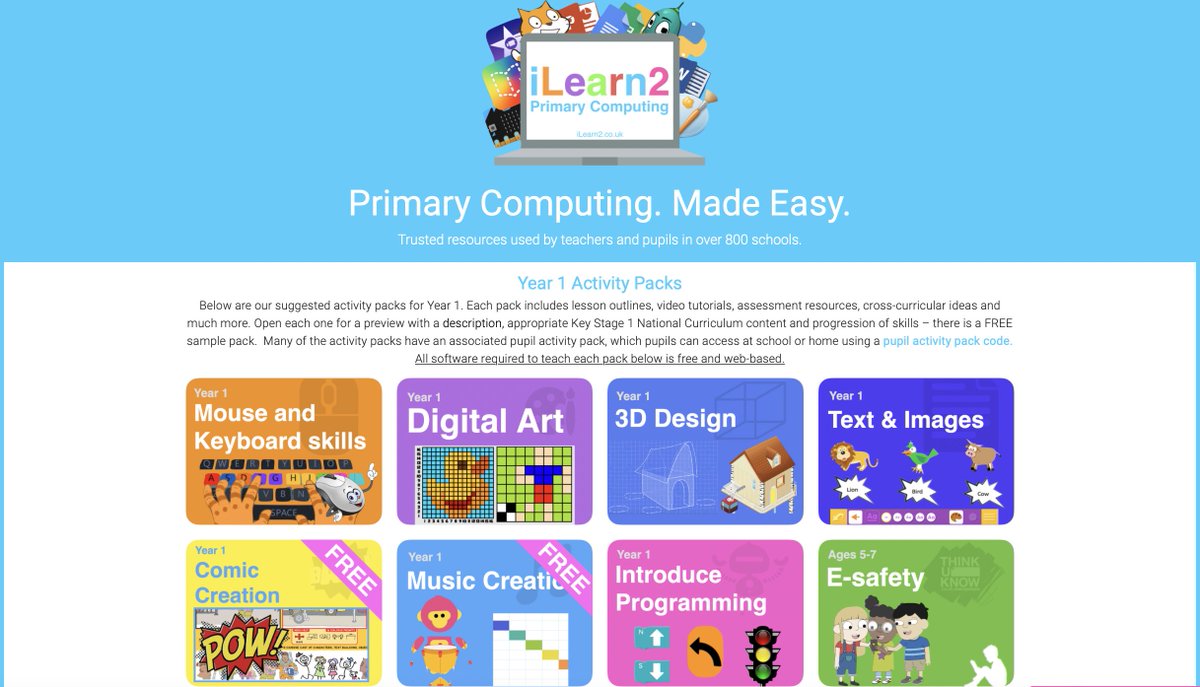Title: "Primary Computing Made Easy: Trusted Resources for Teachers and Pupils"

Caption: 
Discover a comprehensive suite of Primary Computing resources designed to simplify and enhance the learning journey for both teachers and pupils. Featuring a light blue theme, these Year One activity packs encompass various subjects and skills, each aligned with the Key Stage 1 National Curriculum. Delve into topics such as mouse and keyboard skills, digital art, 3D design, text and images, comic creation, music creation, and introductory programming, all tailored for children aged 5 to 7. 

These meticulously crafted packs include lesson outlines, video tutorials, assessment resources, cross-curricular ideas, and detailed progression skills. Each pack also provides a free sample and is accompanied by a pupil activity pack, accessible from school or home via a unique code. All required software is web-based and available at no cost. Explore and preview the resources to find the perfect fit for your classroom needs and unlock the potential of primary computing with trusted and easy-to-use materials.

(Note: The trusted Scratch Cat symbol and various computing icons highlight the engaging and interactive elements of these resources.)